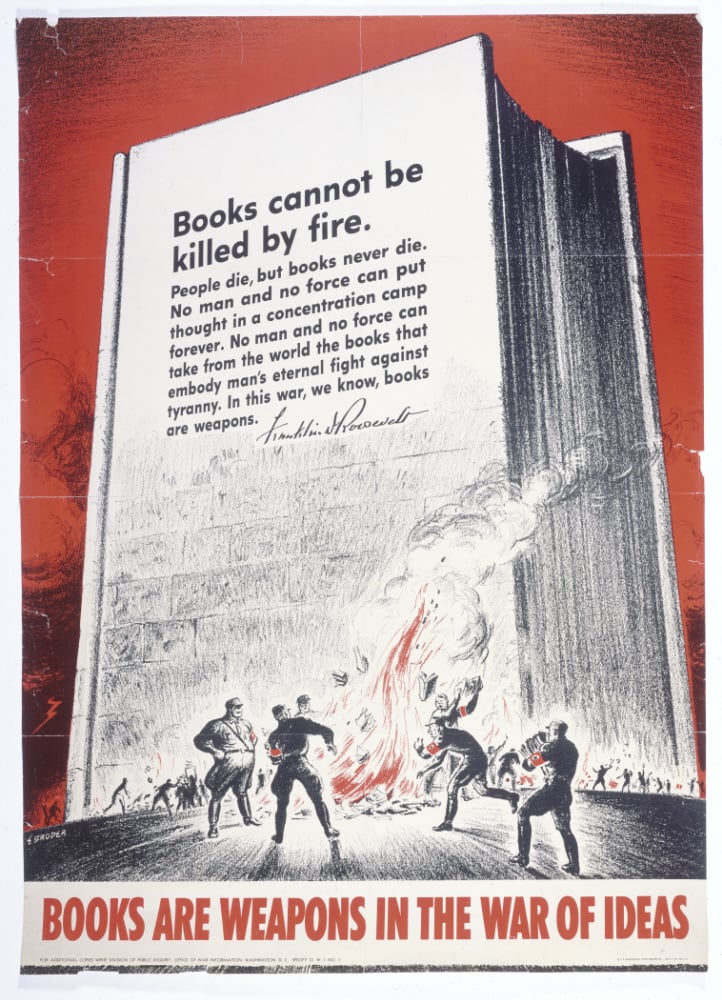The image depicts a powerful World War II-era propaganda poster emphasizing the resilience and indomitable spirit of literature. Central to the black-and-white illustration is a massive book, its bottom half illustrated as if constructed from bricks, suggesting its formidable strength. The book bears the prominent message: "Books cannot be killed by fire, people die, but books never die. No man and no force can put thought into a concentration camp forever. No man and no force can take from the world the books that embody man's eternal fight against tyranny. In this war, we know books are weapons," signed by Franklin D. Roosevelt. 

Flames lick at the base of the book while Nazi soldiers, supervised by a stern military officer, toss more books into the fire, reflecting the historical context of book burnings during the totalitarian regime. The background behind the book is ablaze in red tones, symbolizing a world on fire. At the very bottom, in bold red letters against the stark white background, the poster declares: "Books are weapons in the war of ideas."